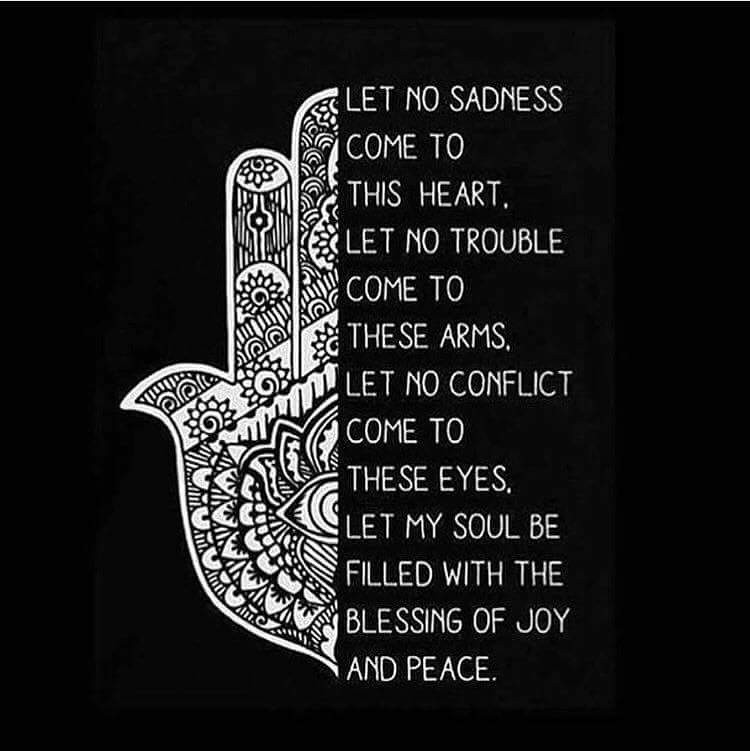The image is a black graphic resonating with the style often seen on social media platforms like Facebook or Instagram, featuring inspirational or philosophical text. The left side of the image boasts a detailed, intricate floral design resembling a henna art pattern, with swirling filigrees, circular shapes, spirals, stars, and flowers. This design evokes the impression of a hand, with the thumb, pointer, and middle fingers prominently depicted, and includes the partial portrayal of an eyelid, all bisected vertically. On the right side of this split design, white text unfolds a mantra or poem which reads: "Let no sadness come to this heart. Let no trouble come to these arms. Let no conflict come to these eyes. Let my soul be filled with the blessings of joy and peace." The text is carefully positioned with a left alignment, contributing to the harmonious and visually appealing composition of the overall graphic.